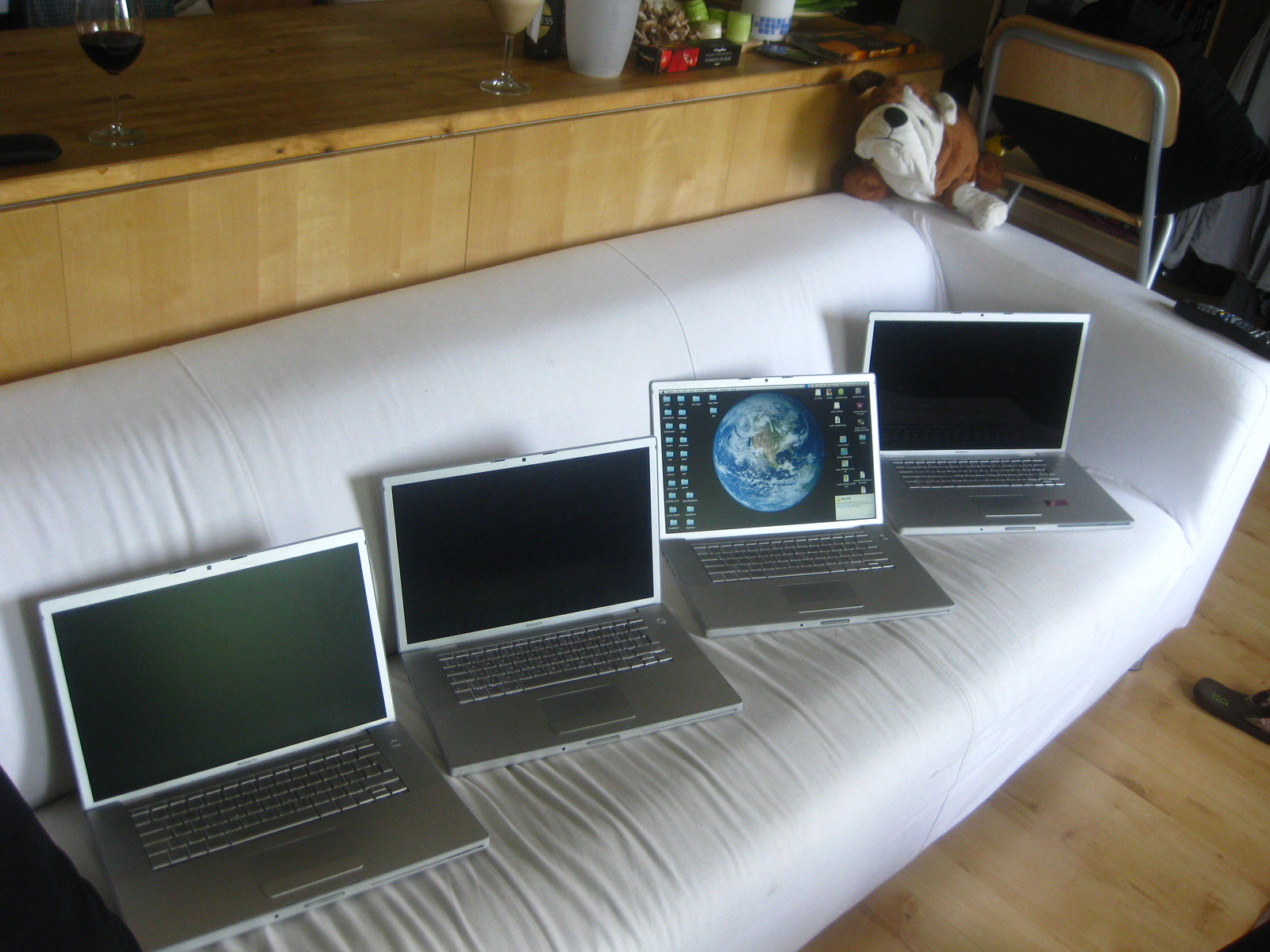In the image, a white couch with a neatly tucked slipcover hosts four silver laptops, all open. The first two and the last one have black screens, while the third displays a galaxy-themed wallpaper featuring Earth against a black background with file icons. Perched in the right-hand corner of the couch is a brown and white stuffed English bulldog. Adjacent to the couch is an Ikea bar-height folding chair with a black pillow on it. Behind the couch stands a light wooden sideboard adorned with various items: a wine glass filled with a dark drink, a partially visible second glass with liquid, and several miscellaneous articles including a cup and a vase fragment. A person's foot is visible in front of the couch. The wooden floor mirrors the sideboard's hue, adding to the room's cohesive aesthetic.